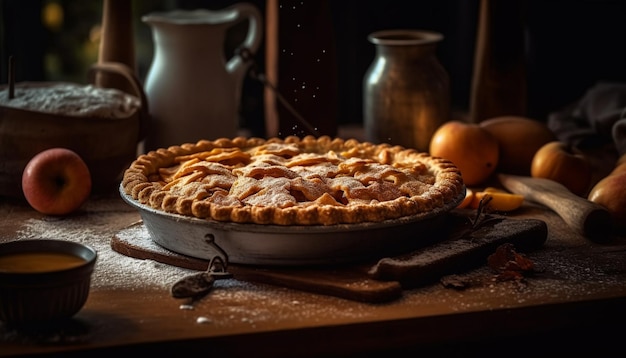The image showcases a freshly baked apple pie, golden brown and adorned with white powdered flour, seated in a vintage silver round pan. The pie features multiple curved edges and visible slices of baked apples at the center. This ensemble rests on a wooden cutting board, all placed on a brown wooden table, giving a rustic, old-world charm to the scene. Flour is scattered on the surface of the table, adding to the lived-in atmosphere of a vintage kitchen. To the left of the pie, there is one apple, while three more apples are arranged on the right side of the table. In the blurred background, a variety of items can be seen: a basket filled with flour, a bowl with a brown liquid, and large metallic pitchers or drink containers, alongside other indistinct fruits, possibly oranges or more apples. The overall setting evokes the warmth and homeliness of an old-fashioned kitchen, reminiscent of a scene from a country magazine.